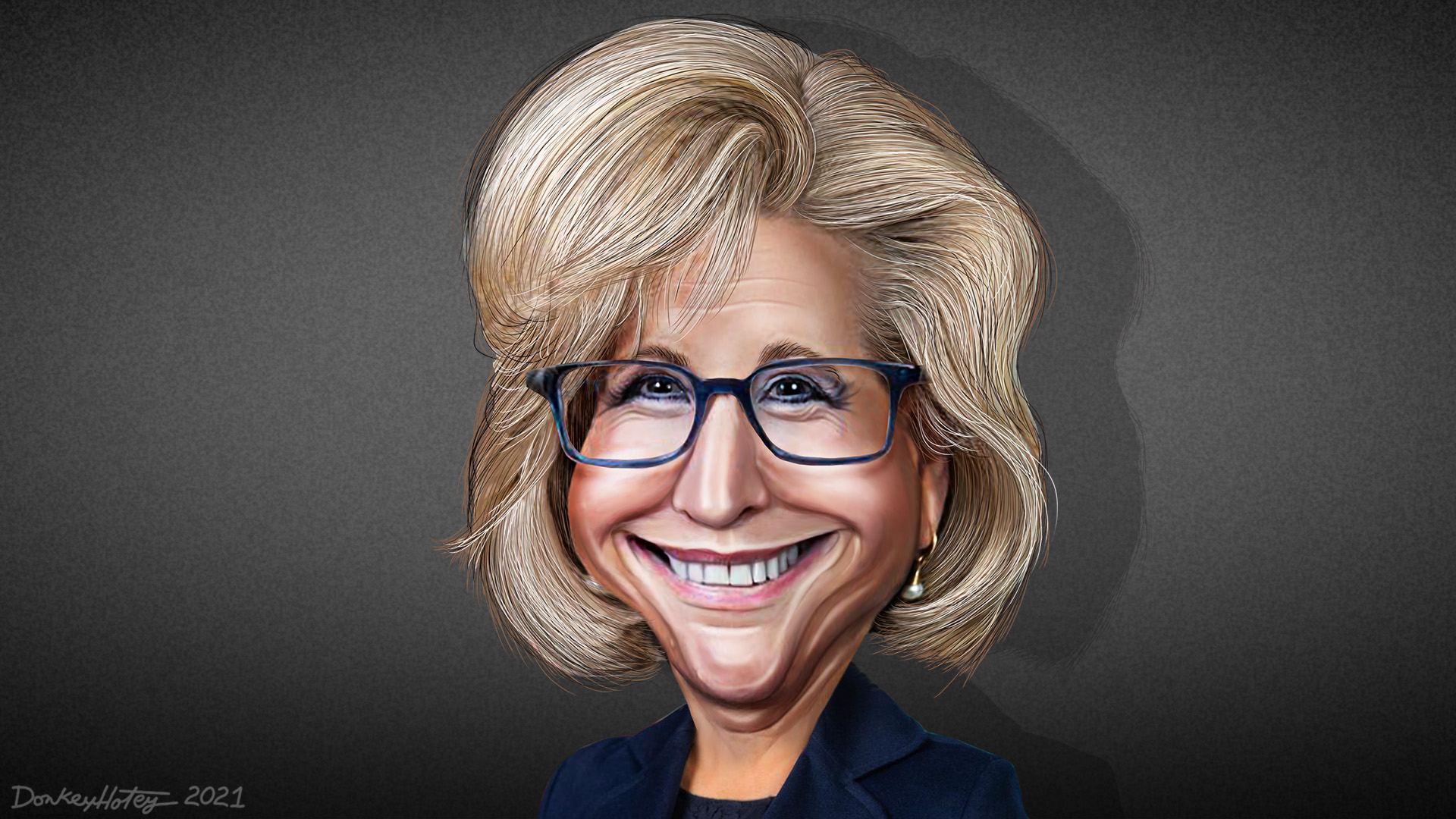This digital artwork is an exaggerated cartoon caricature of Congresswoman Liz Cheney. The piece features her with a comically oversized, elongated head and noticeably large cheeks, all framed by voluminous, wavy blonde hair styled into a bob that curls under at her chin. She sports a huge grin, revealing her top row of teeth, and is adorned with oversized blue glasses, accented by blue eyeliner. She is outfitted in a blue blazer over either a blue or black shirt, with the neckline of the shirt distinctly curled. Completing her attire are what appear to be gold earrings with pearl drops. The background of the image is predominantly gray, with darker shades creating a subtle shadow effect behind her head to the right. The bottom left corner of the image bears the signature "Dookie Hoty 2021" in a white-gray font.